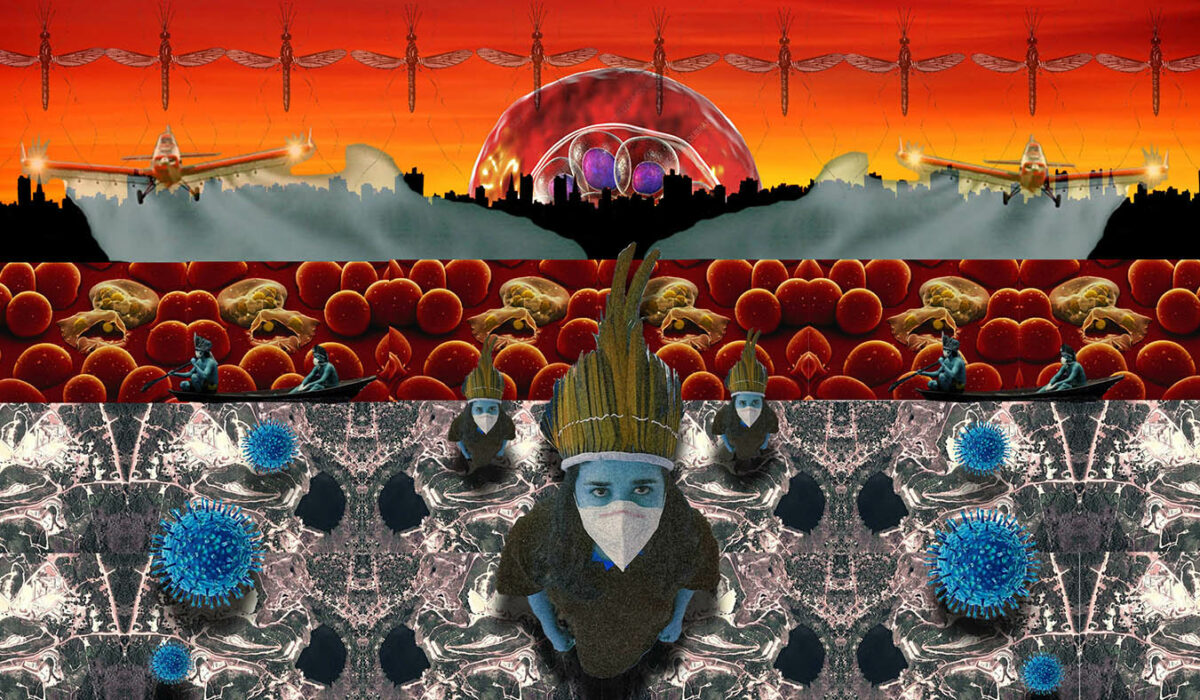The image is a vibrant, digital photo collage divided into three distinct sections, with repeating horizontal patterns and a strong, psychedelic aesthetic. The focal point of the bottom section is a woman, possibly a white female, whose skin is artificially colored blue. She has long, dark hair and wears a white surgical mask reminiscent of those used during the COVID-19 pandemic. Her attire includes a black shirt and a striking headdress composed of feathers in shades of yellowish-orange, black, gray, and even some blue-tipped brown feathers, giving it a Native American appearance. Surrounding her are various geometrical shapes in black and white, interspersed with blue circles adorned with sprout-like extensions.

Above her, there's a row showcasing red, circular forms, possibly representing blood cells or the COVID virus, flanked by two people rowing a black boat, who also have blue skin. This row includes additional blue and yellowish organic forms. Higher still, another row highlights dragonflies arranged wingtip to wingtip, their bodies vertically aligned and wings spread horizontally across a background that fades into warm reds and yellows.

Further elements such as a prominent red circle that could be interpreted as a sun or moon set against a silhouetted cityscape also contribute to the image's layered complexity. Additionally, there are two airplanes approaching the viewer, situated on either side of the red circle, adding to the collage's dynamic, almost surreal composition.